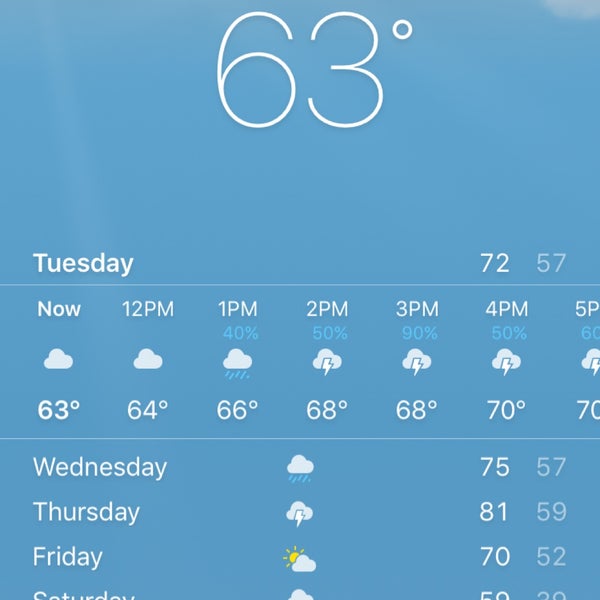A screenshot from the iPhone Weather app with a light blue background. At the top, in white text, it displays "63°F." Below this, the day "Tuesday" is shown with a thin white line underneath. The hourly forecast for the day includes the following times: "Now," "12 PM," "1 PM," "2 PM," "3 PM," "4 PM," and "5 PM," indicating the cloudiness for each hour. 

The chance of rain starts at 40% at 1 PM, increases to 50% by 2 PM, peaks at 90% at 3 PM, then decreases to 50% at 4 PM, and 60% at 5 PM. There are also chances of thundershowers from 2 PM to 5 PM. Corresponding temperatures for these times are: 63°F (Now), 64°F (12 PM), 66°F (1 PM), 68°F (2 PM), 68°F (3 PM), 70°F (4 PM), and 70°F (5 PM). 

A second thin white line separates this section from the next, which lists the following days: "Wednesday," "Thursday," "Friday," and a partially visible "Saturday." The weather is forecasted to be rainy on Wednesday, thundershowers on Thursday, partly cloudy on Friday, and cloudy on Saturday. The temperature range for Wednesday is 75°F to 57°F.